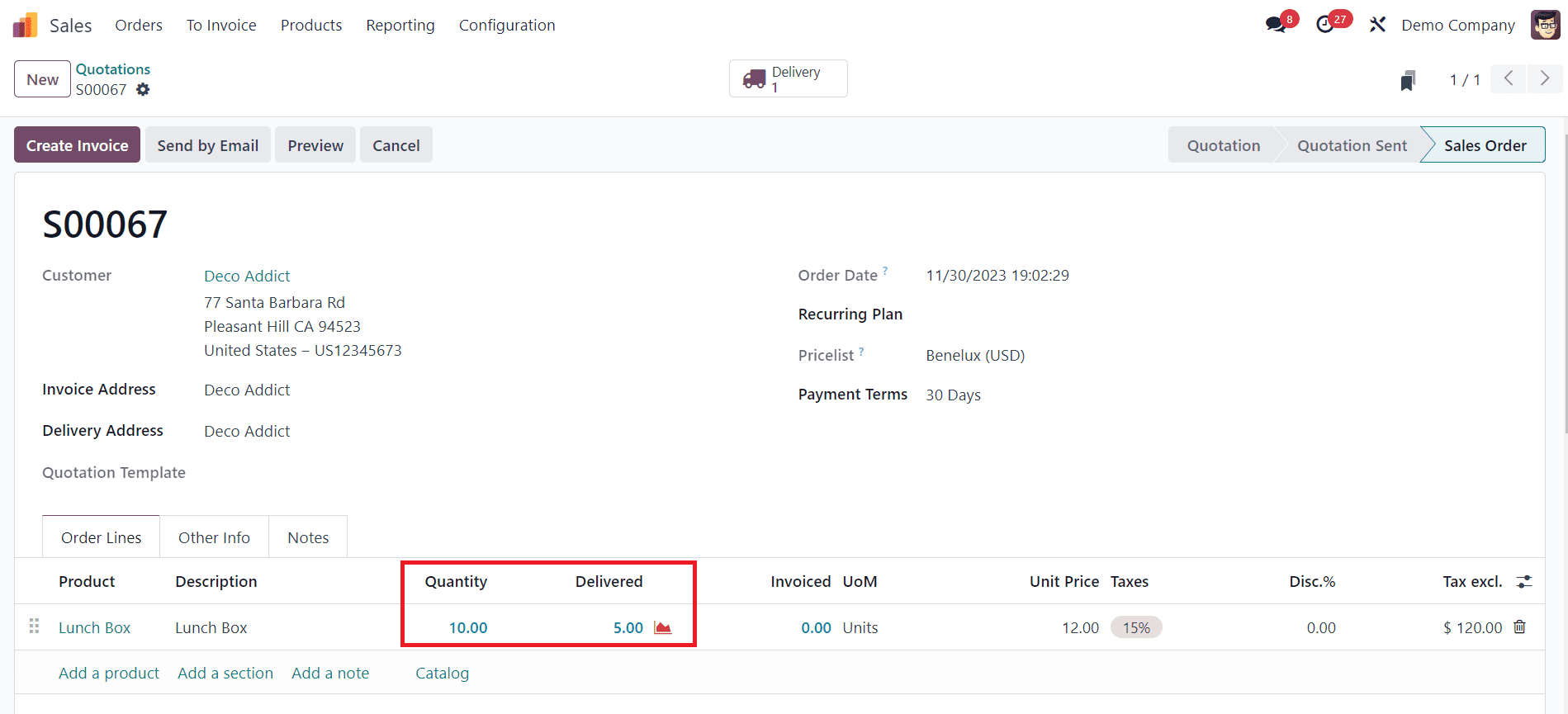This is a detailed and cleaned-up caption for the provided scenario:

---

A screenshot captured from a computer screen showcases a comprehensive web page layout, most likely related to e-commerce or business management. The top navigation bar features menu items labeled: "Sales," "Orders," "To Invoice," "Products," "Reporting," and "Configuration." An icon representing three rectangular boxes in purple, red, and yellow is adjacent to the "Sales" label. 

On the right-hand side, a message icon is marked with the number 8 in a red circle, and a clock icon indicates the number 27 in a red oval. The page header displays the name "Demo Company" accompanied by a square profile picture of a cartoon man wearing glasses. 

Centrally positioned on the page is a rectangular button labeled "Delivery 1," featuring a small drawing of a purple truck. Nearby, a prominent purple button labeled "Create Invoice" in white stands out. All additional text is presented in black and blue.

The customer, named "Deco Addict," has specified sections for their address, invoice address, delivery address, order date, recurring plan, price list, and payment terms. At the bottom of the page, there is a product section detailing an order for a lunch box, including its description, quantity, delivered units, and the total price inclusive of taxes.